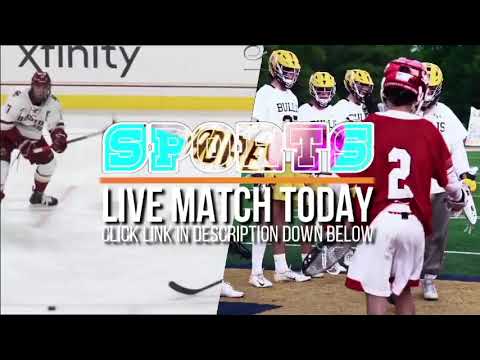The image appears to be a promotional screenshot for live sporting events on a video hosting website. The layout is split into two pictures. The left side showcases a hockey game featuring a player in a white jersey with red gloves, pants, and helmet, holding a hockey stick with a puck in the bottom left corner of the ice rink. The right side features a lacrosse match, where a group of players in white jerseys and yellow helmets is visible. One prominent player facing away from the camera wears a red jersey with the number 2, red helmet, and white shorts. The center of the image displays bold text in a Tiffany blue color that reads "Sports Live Match Today. Click link in description down below," set against a black background border. The imagery on the right includes suggestions of a football or soccer field, adding to the vibrant mix of athletic activities depicted.